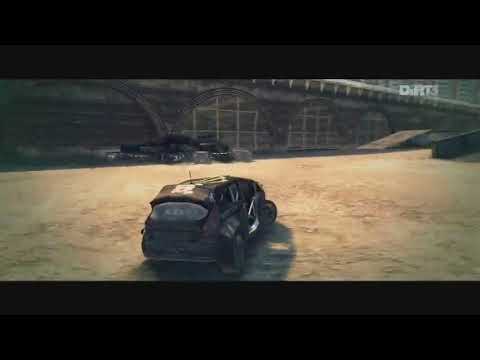The image appears to be taken through a window or an opening with a black horizontal band on both the top and bottom edges. The scene is an illustration, not a photo, showcasing a dirt-filled arena with a race car prominently in the center. The car, viewed from the back, seems slightly beat up and has its front wheels sharply turned to the right. It is black with possibly gold markings or characters on it, with hints of the word "dirts" visible in the upper right corner. In the background, there's another car and a ramp rising to the right, partially obscured. The background is quite dark, revealing some gray structures that might be buildings or scaffolding, with white windows visible. The overall setting feels like a desert-like area with elements suggesting a racing track and large hangar-like doors.